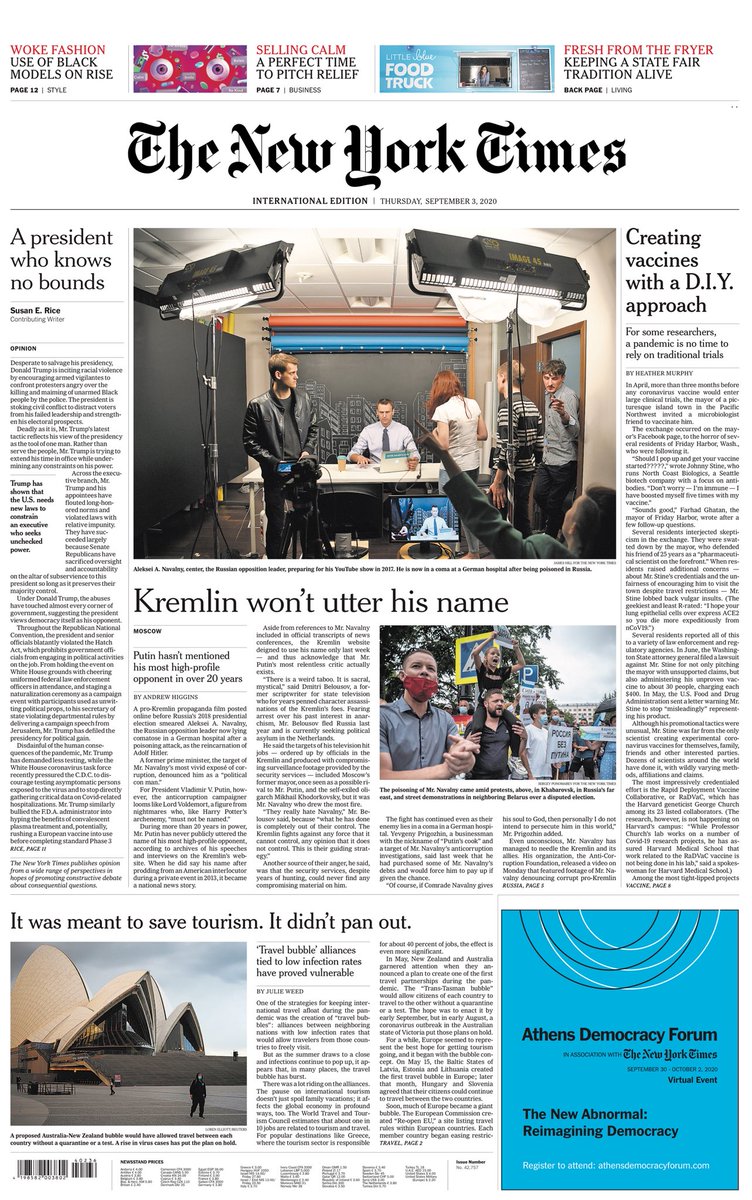This image appears to be a detailed screenshot from the New York Times International Edition, dated Thursday, September 3, 2020. At the top-center, the iconic New York Times logo is prominently displayed alongside the publication date. 

Above the main articles, there are two notable images. On the left, a pair of somewhat cartoonish eyes framed with red and grey hues reflects a stylized approach to illustrating a headline that reads, "Woke Fashion: Use of Black Models on Rise." To its right, another picture features a woman in blue standing near a food truck named "A Little Something Food Truck," accompanied by the headline, "Fresh from the Friar: Keep a State Fair Tradition Alive."

In the center of the page, there is a crucial photo depicting men standing in what resembles a studio setting, illuminated by bright lights. The accompanying headline reveals the details: "Arkhil A. Navaree, creator of the Russian opposition leader, preparing for his YouTube show in either 2017 or 2012." This individual is currently in a coma at a German hospital after being poisoned in Russia. Beneath this, a sub-headline states, "Kremlin Won't Utter His Name."

To the left of this centerpiece image, another major headline reads, "A President Who Knows No Bounds," while on the right, another article is entitled, "Creating Vaccines with a DIY Approach."

Further down, a headline declares, "It Was Meant to Save Tourism, It Didn't Pan Out," alongside an image of the Sydney Opera House. The bottom right corner of the page features an advertisement with a blue background for the Athens Democracy Forum, highlighting the theme "The New Abnormal: Reimagining Democracy."

Due to the dense text and small font size in certain sections, some additional details remain difficult to discern.